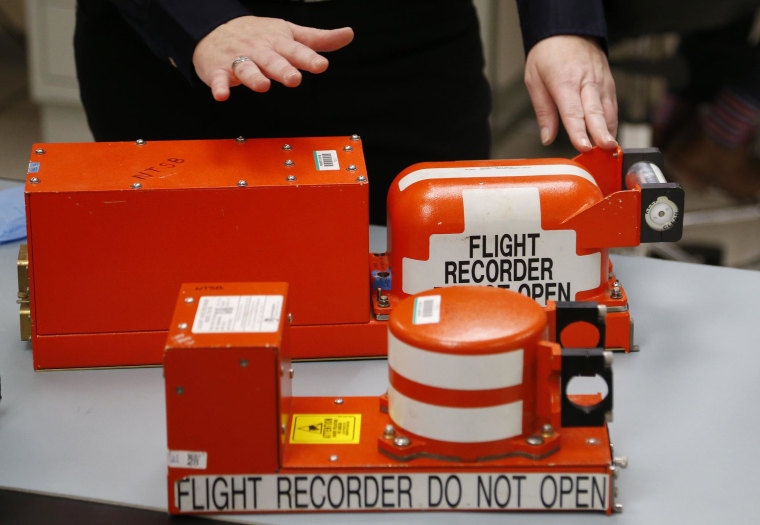In the image, a person dressed in a long-sleeve black outfit demonstrates a flight recorder, commonly known as a black box, although it is actually a shiny red. Only the person’s hands are visible, adorned with a ring on the right ring finger, gently touching or hovering over the flight recorder. The black box prominently displays the text "Flight Recorder Do Not Open" in black lettering over a white background. The larger, rectangular main unit features various labels, including "NTSB" and barcodes, with screws visible on its surface. A smaller, similarly labeled flight recorder is positioned in the foreground, consisting of a metal housing with a cylindrical component attached to the right. Both devices are placed on a gray countertop structure, possibly a table or cabinet. The scene is well-lit and detailed, giving a clear and realistic view of the newer-looking, unworn equipment. The red of the flight recorders is notably vibrant, capturing attention against the neutral background.